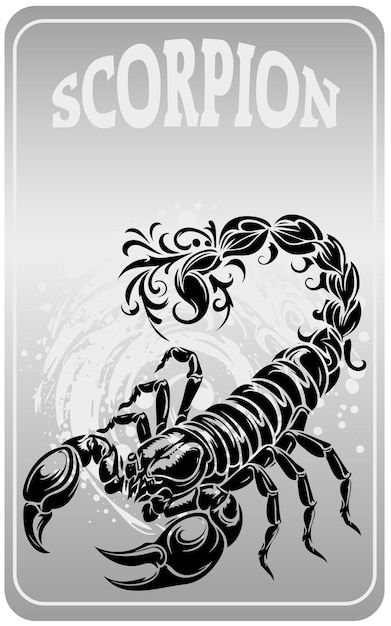The image is a detailed drawing of a scorpion prominently displayed on a light gray background with rounded corners, trimmed with a white line. The scorpion itself is black with menacing claws, three legs on each side, a detailed mouth, and a long, bumpy, elongated body and tail adorned with vine-like decorations that resemble curls and leaves towards the stinger. The word "Scorpion" is featured at the top in white capital letters, which start smaller, enlarge towards the middle, and then decrease in size. Behind the central scorpion figure, there is a white circular patterned design composed of circles within circles and dotted embellishments. The overall style of the image resembles that of a playing card, poster, or informational sign, with the scorpion centrally positioned against the gray backdrop.